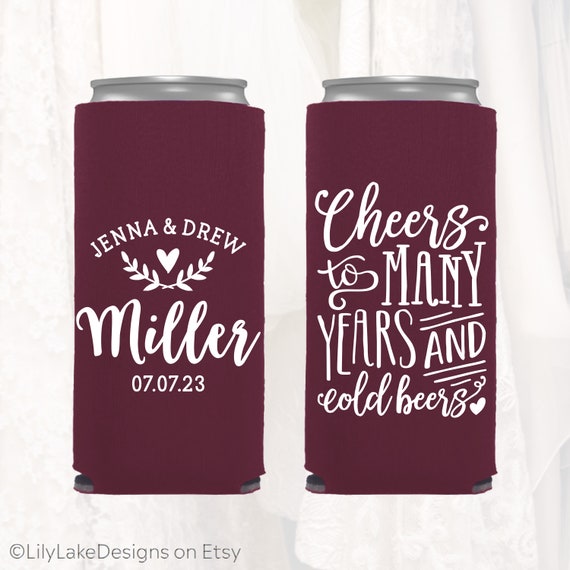This photograph features two 16-ounce beer cans nestled in maroon foam koozies, designed to keep the beverages cold. The can on the left reads "Jenna and Drew Miller 07.07.23" in bold, white, stylized letters with additional decorative elements like a heart and leaves. The can on the right declares "Cheers to many years and cold beers" in a similar white font, accompanied by a small heart. Both cans are set against a grayish-white, mottled background, evoking a cartoonish style. In the lower left corner, "Lily Lake designs on Etsy" is subtly printed in gray, likely indicating the source of these custom-designed koozies, which celebrate a special occasion, presumably Jenna and Drew's wedding.